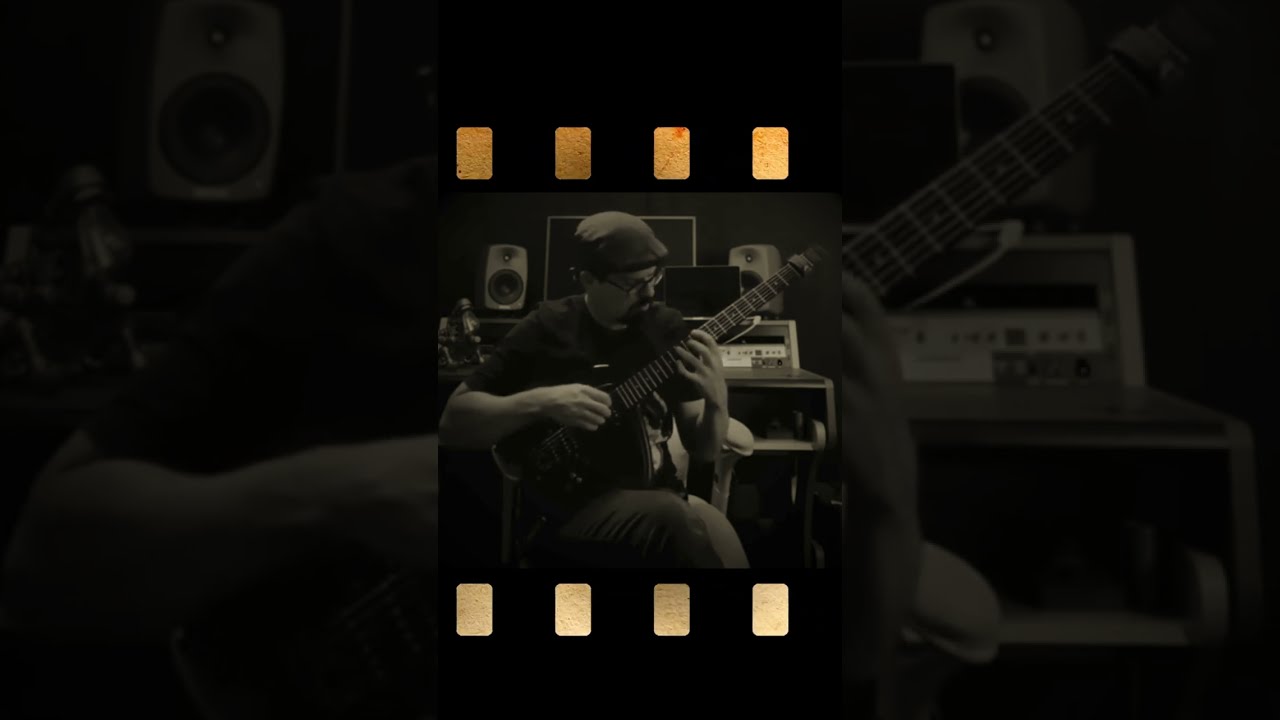In this evocative black and white photograph, a bearded Caucasian man with sunglasses is captured playing a black guitar. Seated with his legs crossed on a chair in a recording studio, he is deeply focused, staring down at his instrument. The man is adorned in dark clothing, including a black cap, t-shirt, and pants. Behind him, a desk hosts a computer monitor flanked by white speakers. The setting is accentuated by a black wall, which is adorned with four glowing yellow rectangles above the computer monitor and four pale yellow rectangles at the bottom of the image. The overall composition of the photograph includes a zoomed-in background that showcases the man's arms and guitar, further emphasizing the intimate atmosphere of his creative space.